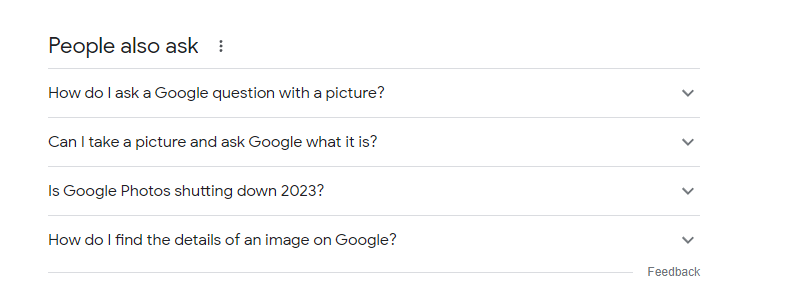The image is a screenshot from a website displaying a "People also ask" section, set against a white background. At the top, "People also ask" is written in larger text with the initial "P" capitalized, followed by three vertically stacked dots. 

Below this heading, a thin horizontal line separates it from a series of questions, each accompanied by a downward-facing arrow indicating a drop-down menu. The first question reads, "How do I ask a Google question with a picture?" with "Google" capitalized.

A thin line separates this question from the next, which asks, "Can I take a picture and ask Google what it is?" Again, "Google" is capitalized.

Following this is another line, then the question, "Is Google Photos shutting down, 2023?" Here, both "Google" and "Photos" have their initial letters capitalized.

The subsequent question is, "How do I find the details of an image on Google?", with "Google" again capitalized, followed by another downward-facing arrow on the right.

At the bottom of the list, there's a final link labeled "Feedback" with a capital "F." Each question in the list is clearly separated by thin horizontal lines, and the consistent formatting underscores the website's structured layout for user inquiries.